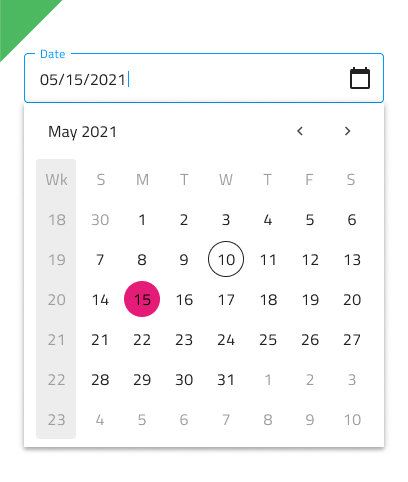The image displays a calendar application interface with a distinctive green triangle pointing towards the upper left corner. Located beneath the triangle is a blue rectangular box labeled "Date," showing the date "05/15/2001" in black text. To the right of this date box is a small calendar icon, presumably a button for accessing different months, though its specific functionality is uncertain.

Below this setup, "May 2021" is prominently displayed in black text, flanked by navigation arrows—a less than sign (<) for scrolling back to previous months and a greater than sign (>) for advancing to future months. The calendar itself features a white background, with black text marking the various elements.

On the far left of the calendar, extending vertically from top to bottom, is a column labeled "WK," indicating the weeks numbered from 18 to 23. Across the top, from left to right, the days of the week are denoted by their initials: SMTWTFS (Sunday through Saturday). The calendar grid starts with Saturday, the 30th of April, and continues sequentially, with Monday being the 1st of May, Tuesday the 2nd, and so forth, up to the 10th of June, although the month of June itself is not labeled.

Significant dates are marked with circles: a clear circle around the 10th and a filled pink circle around the 15th, highlighting the selected date "05/15/2001."

Overall, the interface offers a clean and functional layout, with essential features easily accessible for users to manage their schedules effectively.